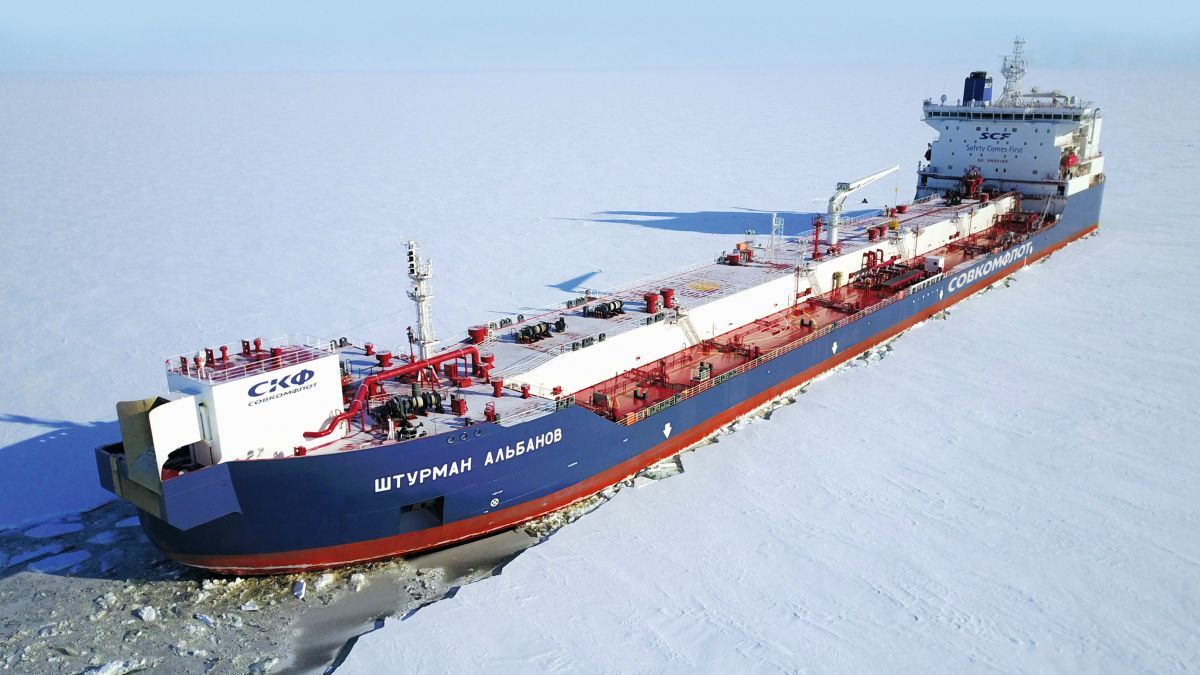This image captures a large, intricate icebreaker or cargo ship navigating through a frozen lake or sea, likely in a very cold region. The towering vessel, predominantly colored in shades of red, white, and navy blue, dominates the frame from the bottom left to the top right. With Cyrillic writing on its side, suggesting it is of Russian or Ukrainian origin, the ship appears to be performing the vital task of cracking a path through the icy expanse. The forefront features a tall tower, multiple cranes, and a network of pipes, emphasizing its robust and complex engineering. The ship cuts through the ice, creating visible cracks on either side and casting elongated shadows behind and in front of it as it heads away to the right. Its operation and imposing structure paint a picture of strength and purpose amidst the stark, frozen backdrop.